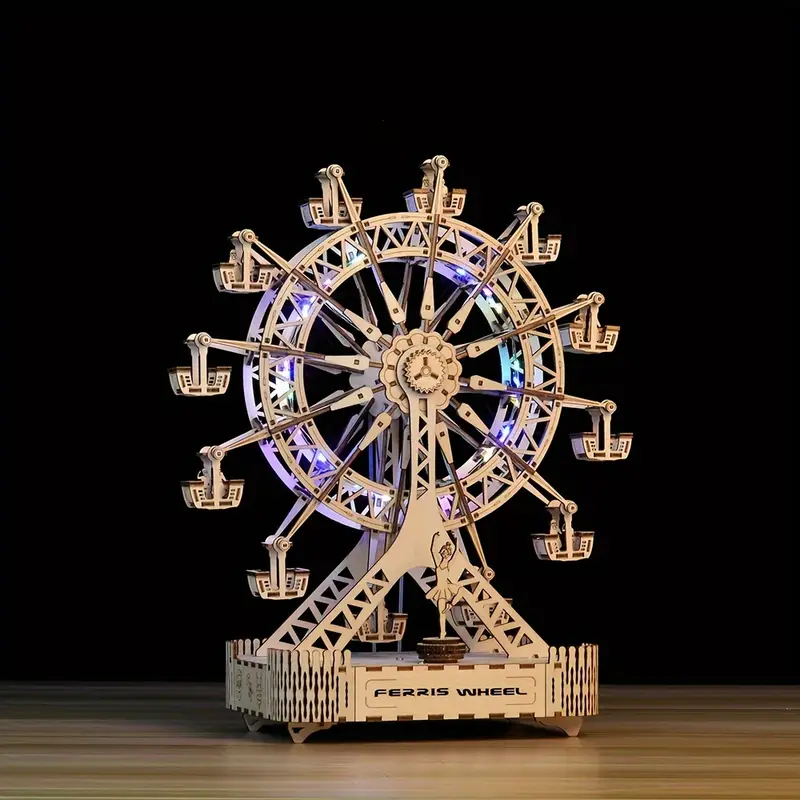This detailed image showcases a 3D laser-cut model of a Ferris wheel meticulously assembled from a thin, possibly balsa wood material. The model features intricate details like a tiny gate cutout and a three-sided foundation that supports the structure. Delicate score and etch marks from the laser cutting process are visible, further highlighting its handcrafted nature. The Ferris wheel itself is adorned with colored lights—primarily blue, turquoise, purple, and white—that illuminate its circumference. Hanging from the wheel are 12 to 13 miniature baskets where patrons would typically sit. The entire model rests on a wooden surface, set against a stark black background that accentuates its intricate craftsmanship and vibrant lighting.